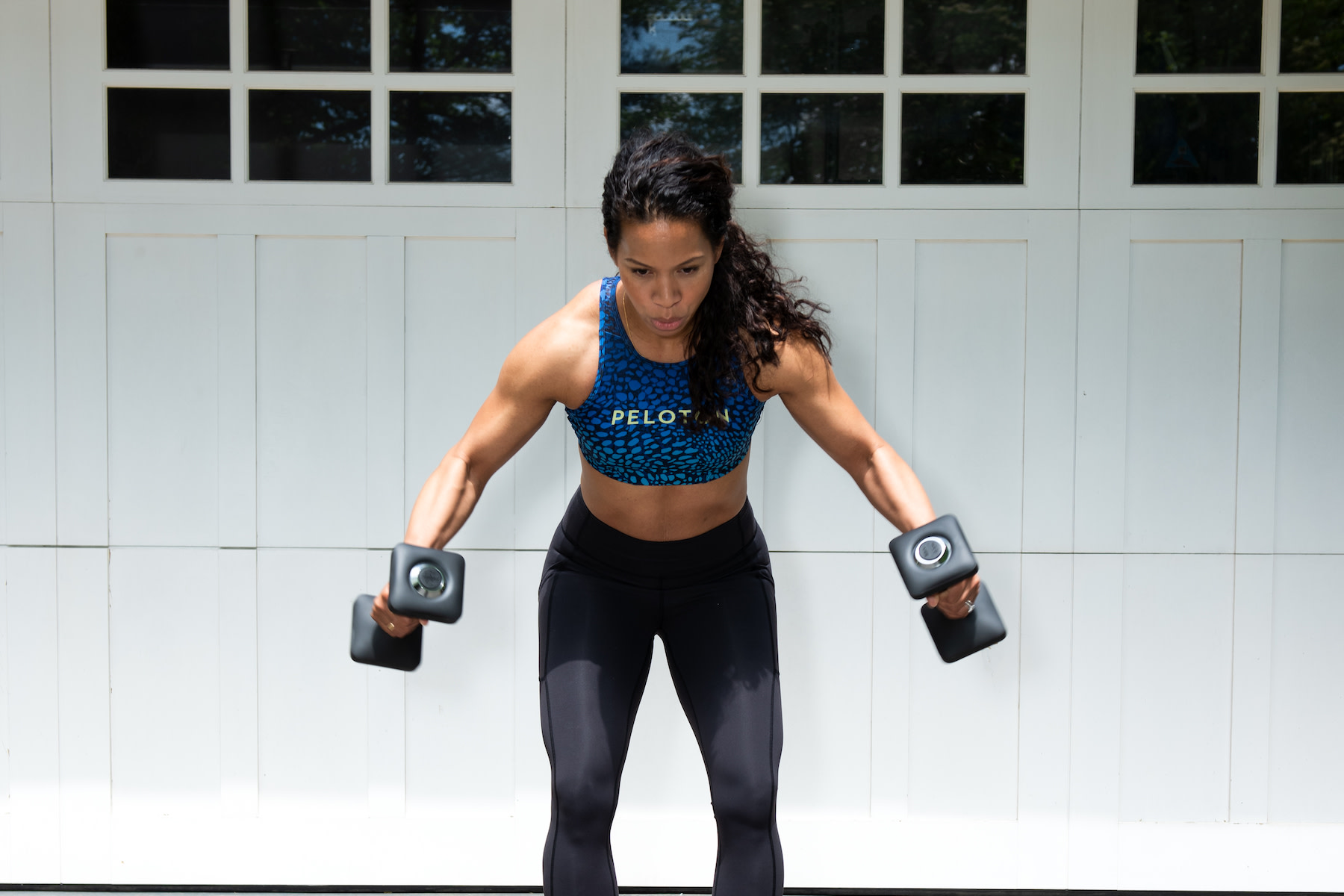In this photograph taken outdoors, a fit woman is performing a workout in front of a white garage door adorned with a series of black windows arranged in two rows of three rectangles each. The image captures her from the calves upwards, focusing on her intense workout pose. She is wearing black, tight sweatpants and a small, blue and black sports bra with the word "Peloton" prominently displayed in white lettering across her chest. Her mocha-colored skin and toned, muscular arms are highlighted as she grips two square-shaped dumbbells in each hand. Her long, dark hair flows over her shoulder, pulled back in a slightly curly ponytail. The expression on her face is serious and focused as she exhales, visibly flexing her muscles while lifting the weights.